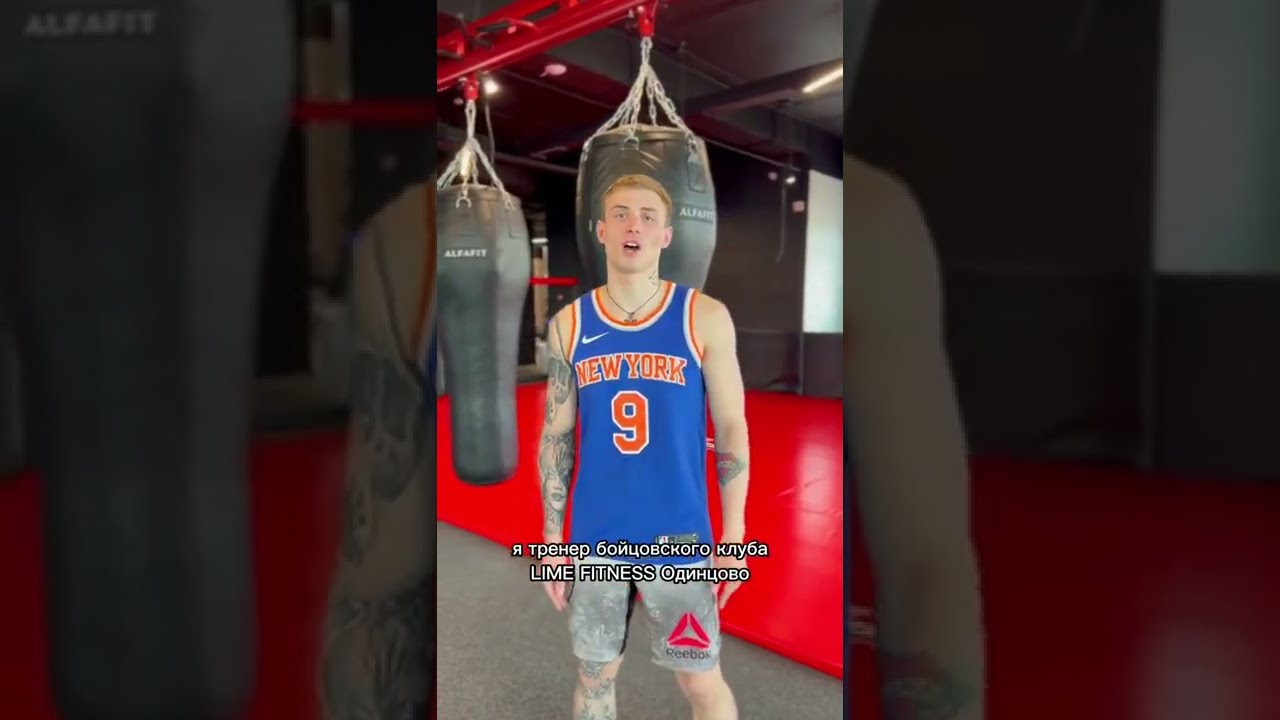The image centers on a young man standing in a gymnasium, bisected by a bright vertical strip with darkened sides. He is wearing a blue Nike tank top emblazoned with "New York" in orange with a white outline, and the number 9 below. His tank top also features a white Nike swoosh on the left chest. He sports light gray Reebok shorts with a black pattern and a red triangle at the bottom, accompanied by the Reebok logo and text. The young man appears to have short blonde hair and is adorned with a necklace. His skin is white, and he’s decorated with tattoos: an elaborate design on his right arm and leg, and a smaller one on his left forearm.

In the background, red mats cover the gym floor, contrasting with the gray mat he stands on. Several black punching bags marked "Alphafit" hang from silver chains attached to metal bars on the ceiling, integrated with the prominent red rafters. Russian text, along with “Lime Fitness,” is overlaid at the bottom of his torso. The man stands facing the camera, slightly open-mouthed, seemingly in the midst of speaking. The overhead lights cast a layered illumination throughout the space, enhancing the vivid details of the gym and his appearance.